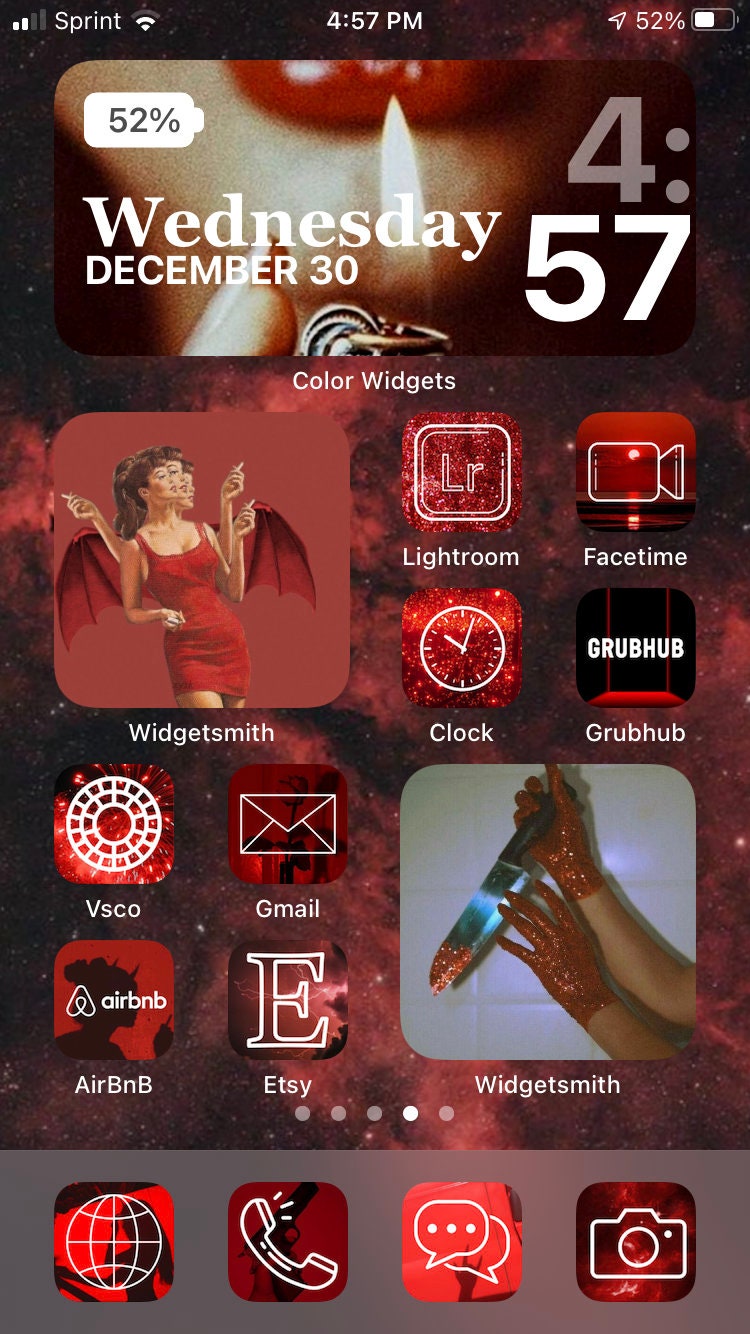The screenshot depicts a smartphone home screen, showcasing a variety of elements and a distinct red and black theme. In the status bar at the top, the device is connected to the Sprint network with two bars of signal strength, two bars of Wi-Fi, the time is 4:57 PM, and the battery is at 52%. The background image of the home screen displays the bottom half of a woman's face with striking bright red lips, accompanied by the date and time: Wednesday, December 30th, at 4:57.

The top left of the home screen features a large widget labeled "Widget Smith," displaying a light pinkish background with a woman in a red dress and red wings. To the right are four app icons: Lightroom, FaceTime, Clock, and Grubhub, all adhering to the red and black color scheme. 

Below these icons is another large Widget Smith image, showing a female hand holding a knife with a glittery red substance, appearing like gloves. Beneath this widget are four additional app icons, though their specific apps aren't detailed. 

At the bottom of the screen are the default navigation icons, including a web browser symbol (world map), phone, messaging, and camera icons.